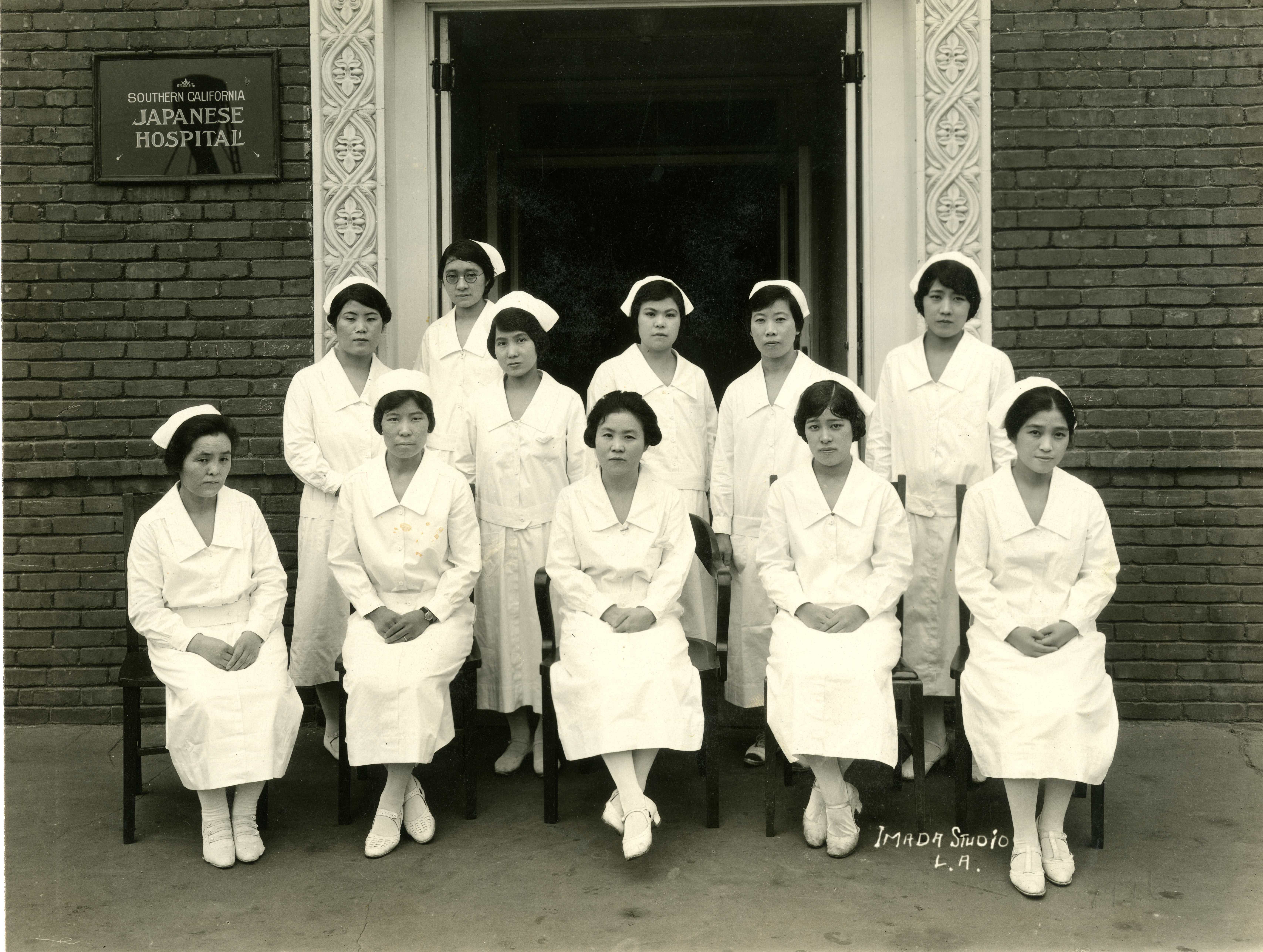This sepia-toned black-and-white photograph captures 11 Japanese nurses posing in front of an entrance, labeled "Southern California Japanese Hospital" in white text within a black frame near the top left. The nurses, all wearing identical white uniforms with long sleeves, collars, white nursing hats (except for two), white stockings, and moderately tall high-heeled shoes, have medium-length black hair. Five nurses are seated in the front row, while the remaining six stand behind them. They are positioned on a plain concrete floor flanked by dark brick walls, with a large door in the background featuring intricately patterned columns. The doorway's interior appears shadowed and somewhat obscured. The bottom right corner of the image bears the mark of "Imada Studio LA," highlighting its historical context.